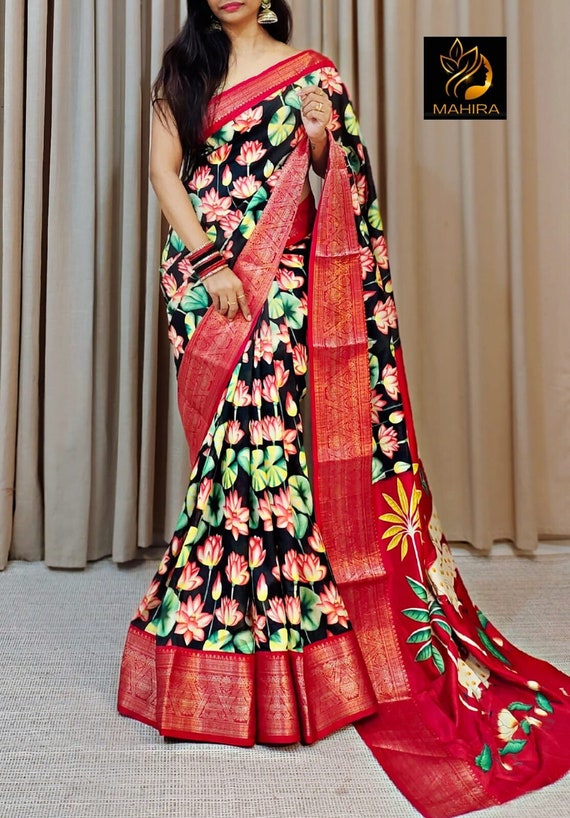In this detailed image, the focus is on the lower portion of a woman standing gracefully. She is wearing an exquisitely long dress that cascades to the gray, carpeted flooring. The hemline of the dress is asymmetrical, with the right side extending longer than the left. The edge of the dress is adorned with intricate designs: predominantly red, featuring green and white leaf-like patterns, alongside a striking yellow flower. 

The dress itself showcases a rich tapestry of design, set against a black background, embellished with clusters of pink flowers, green leaves, and occasional yellow-green blooms, densely interwoven to create a lush, floral pattern. The upper part of the dress is a solid, vibrant red. The woman is shown gently holding a part of her dress with her left hand, while her right hand is elegantly poised over her right shoulder. Her long black hair flows down the left side, adding to her graceful appearance.

In the backdrop, there is a light brown curtain, complementing the scene, along with a prominent square black emblem that reads "Mahira," highlighted by a gold design at its center, adding a touch of sophistication to the overall composition.